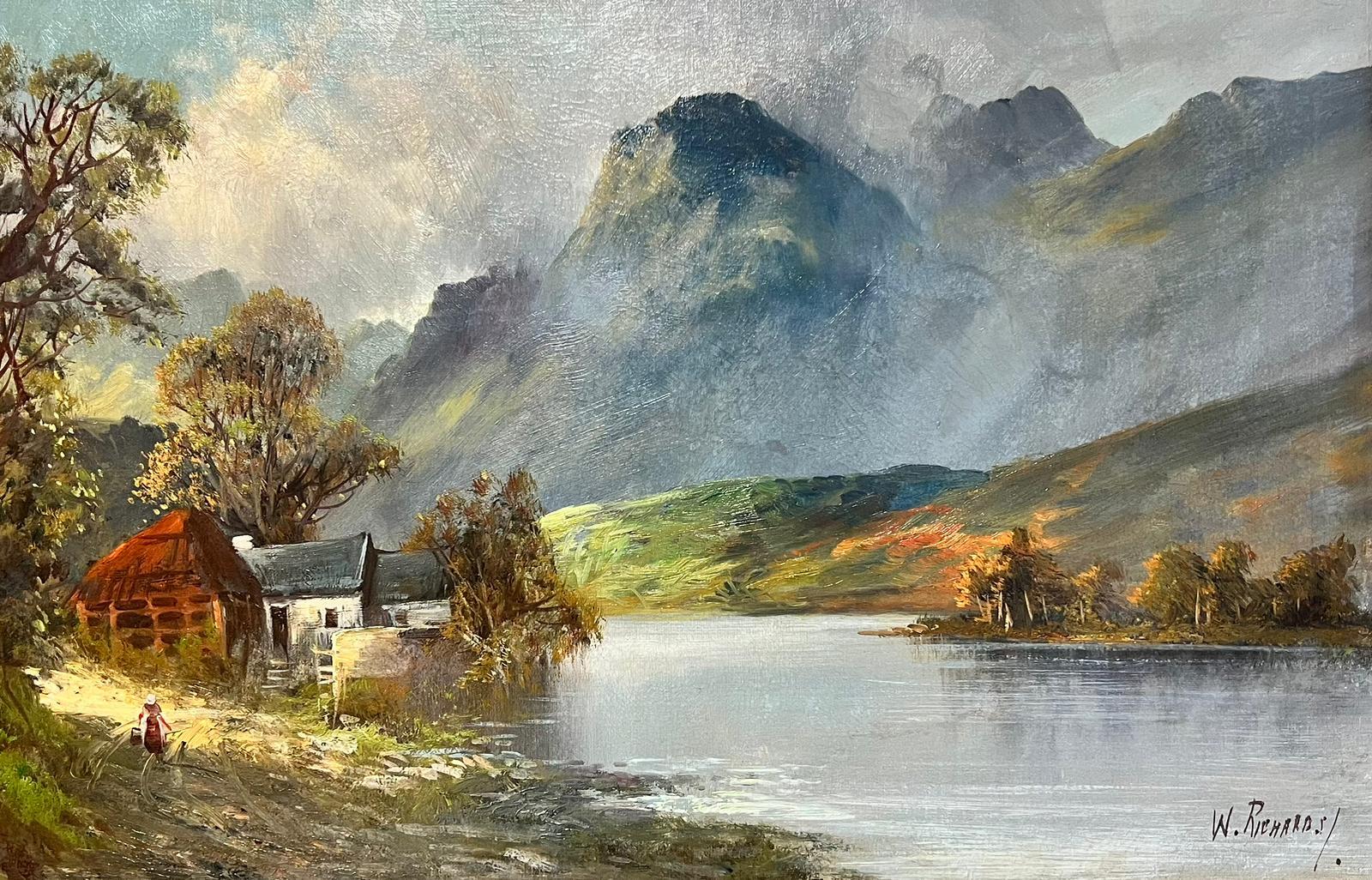The image is a serene landscape painting showcasing a calm, silver-gray pond or small lake, surrounded by lush green grasses and hills. Prominent in the background are dark gray mountains, adorned with hints of dark teal. The scene is overcast with a mostly cloudy sky, evoking a peaceful and untouched natural ambiance. On the left side of the image, there is a striking red house or hut amid the greenery, accompanied by a tree with green leaves. A white structure, possibly a small barn or house, is also visible amidst the grassy area, enhanced by nearby trees. Additionally, to the far left in the lower part of the image, there is a depiction of a person with their arms outstretched, possibly carrying a basket in each hand. The artist, whose name begins with "W-R-I-E-H-A-R-D-S," has signed the painting. The overall composition is horizontally oriented and captures the essence of a tranquil, nature-dominated landscape.